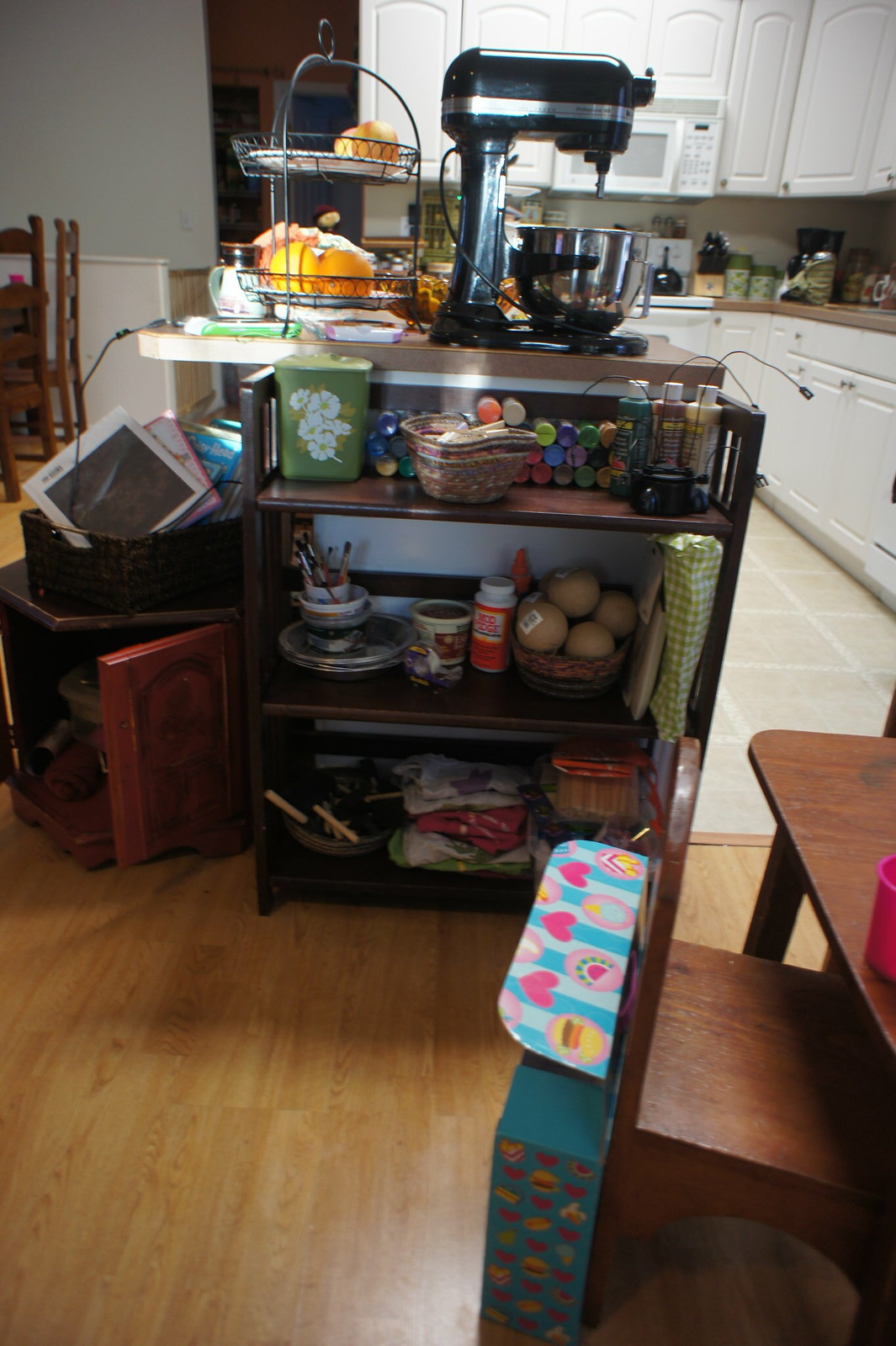The image captures a vibrant and cozy scene in a home, viewed from the dining room into the adjacent kitchen. The foreground features a warm wood floor, with the grain running from the bottom of the image to the top. In the bottom right corner, there is a wooden chair next to a small, reddish wood table. On the table sits a pink cup, adding a splash of color. Behind the chair, a light and dark blue striped box adorned with pink hearts and circles is visible.

Directly ahead, a three-tier shelving unit is prominently displayed. The top shelf, on the left, holds a green canister decorated with flowers and a basket in front of it, alongside horizontally-laid paint bottles. The right side of the top shelf houses a black container brimming with small lights and three large paint bottles. The middle shelf features various dishes, including plates and bowls, a cup filled with paintbrushes, a roll of scotch tape, and several labeled cans and containers. To the right, there is a woven basket containing fruit, and a green-and-white gingham bag. The bottom shelf is cluttered with cloths, brooms, and other miscellaneous items.

To the left of the shelving unit is a quaint seating area, anchored by an octagonal end table with an open door, revealing books, while a basket sits atop the table. Wooden chairs and a baby gate, likely leading to stairs, can be seen in the background, set against a bluish-cream wall.

The kitchen itself features white cabinetry and large beige tile floors. The countertops, a brownish hue, add warmth to the space. At the end of the counter, a black KitchenAid mixer stands tall beside a two-tier pie rack filled with fruit, accompanied by a low glass bottle with a top. Canisters line the back wall, beneath a white microwave that is mounted above the matching stove. A black kettle rests on the stovetop, completing this inviting and bustling kitchen scene.